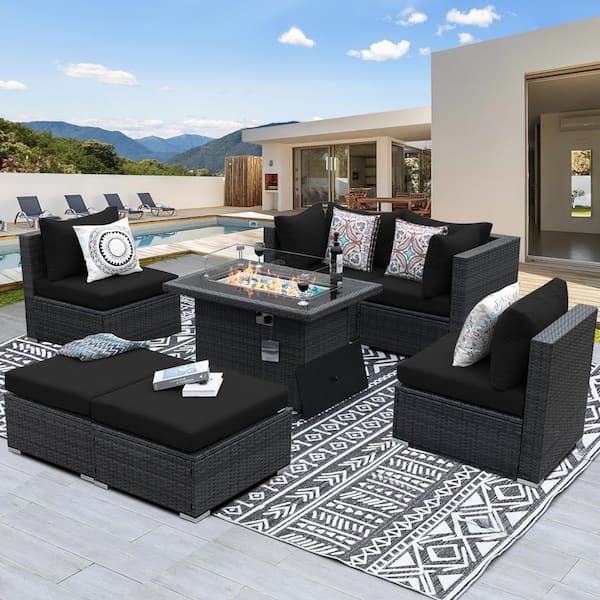The image showcases a stylish patio area set against a scenic background. Dominating the foreground, an arrangement of black rattan furniture occupies a large, geometric-patterned gray and white rug. The setup includes a love seat, two chairs, and a bench, all adorned with black cushions and vibrant throw pillows in shades of gold, blue, and white. A central glass-top coffee table holds a bottle of dark wine and two filled wine glasses, possibly beside a game setup or another decorative element. 

To the side of the seating area, two ottomans are aligned, giving the space more versatility. The patio features a sleek gray floor and, in the middle, a modern fire pit with gas flames dancing among glass rocks. Just beyond, a rectangular swimming pool is bordered by chic gray chaise lounges, inviting relaxation. 

The backdrop reveals part of a modern, one-level house with abundant glass windows and sliding doors, allowing for ample natural light. Enclosing the property is a high beige wall and within the same area, there's an enclosed outdoor shower, adding to the luxurious feel. The scene extends further to capture a panorama of lush green mountain ranges under a clear light blue sky dotted with powdery white clouds, completing the idyllic outdoor setting.